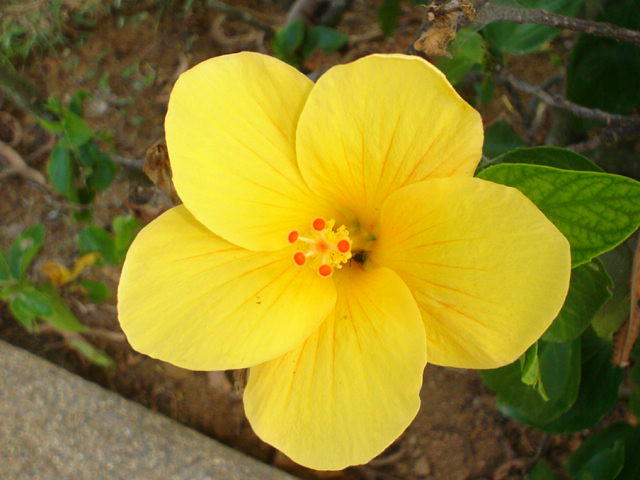This detailed photograph captures a single, vibrant yellow flower positioned at the center of the image, radiating with five broad petals. The flower's core is visually striking, featuring a cluster of stamen with five orange-red dots ready for pollination. Surrounding the flower are lush green leaves, some positioned to the right and left, blending into the backdrop where dirt forms the majority of the ground. A small portion of concrete is visible in the bottom left corner, suggesting this flower might be in a garden or planter. The image focuses intensely on the flower, capturing its beauty amid natural elements, with the earthy brown of the soil and the gray of the concrete adding contrast. The photograph appears to be a personal shot, emphasizing the flower's delicate yet vibrant presence in its natural environment.